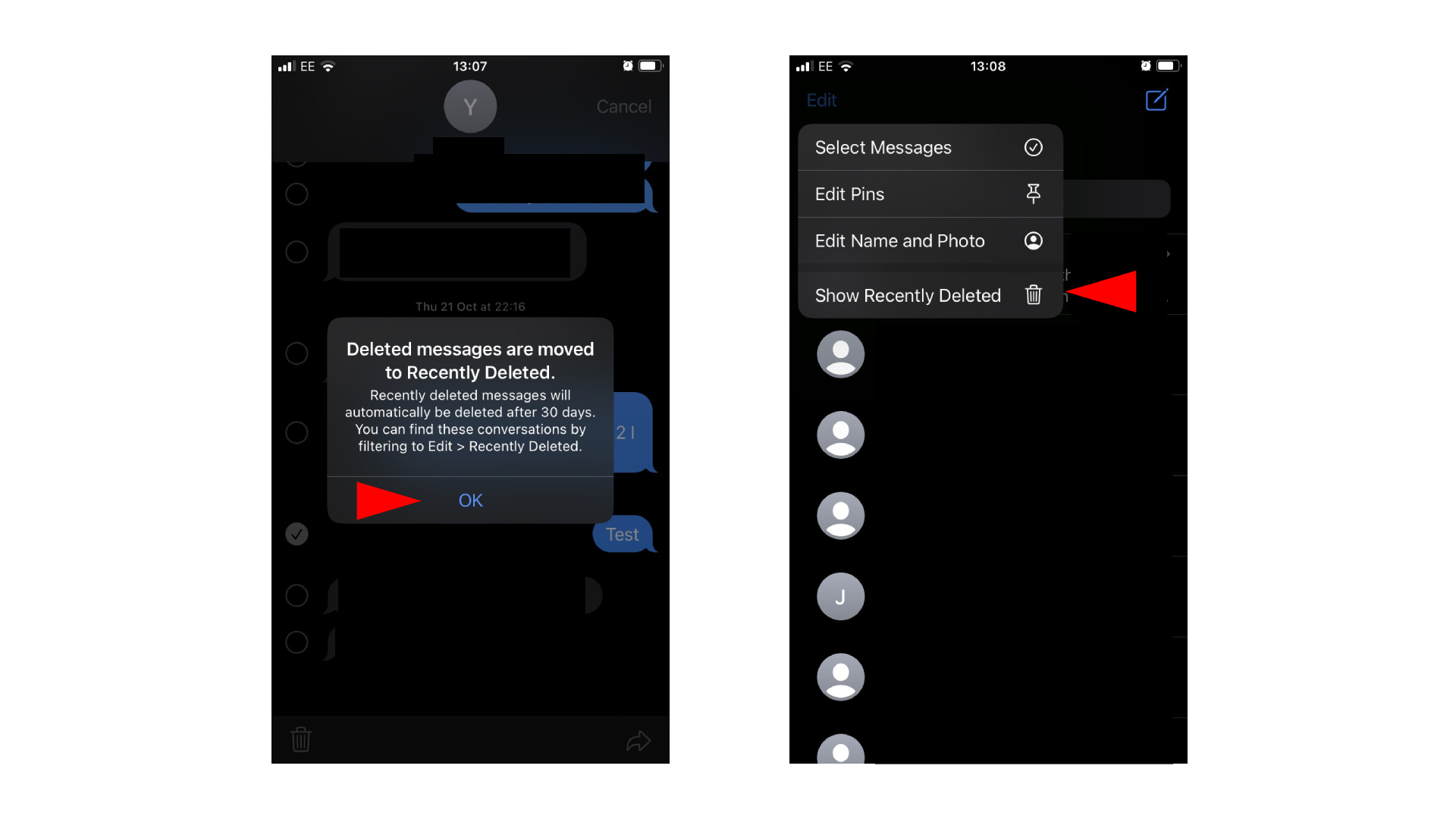The image consists of two side-by-side screenshots taken from a phone, both set against a black background and taken one minute apart, at 13:07 and 13:08 respectively.

In the 13:07 screenshot (left side):
- It shows a text message conversation where the top contact symbol is a grey circle with a "Y", indicating no profile picture.
- The messages in the chat are obscured by black, with a visible fragment reading "test."
- A pop-up menu appears over the conversation, stating:
  "Delete messages. Deleted messages are moved to recently deleted. Recently deleted messages will automatically be deleted after 30 days. You can find these conversations by filtering to edit recently deleted."
- Below this message is a blue button labeled "OK," prominently highlighted by a large red arrow pointing towards it.

In the 13:08 screenshot (right side):
- It shows a list of contacts, most denoted by a generic "empty frame" icon, except for one labeled "J," but all are obscured by black.
- An active menu highlights options such as "Select Messages," "Edit Pins," "Edit Name and Photo," and "Show Recently Deleted," with a large red arrow pointing to "Show Recently Deleted."

The captions should provide a clear and comprehensive below of how to navigate deleting and locating recently deleted messages on a phone.